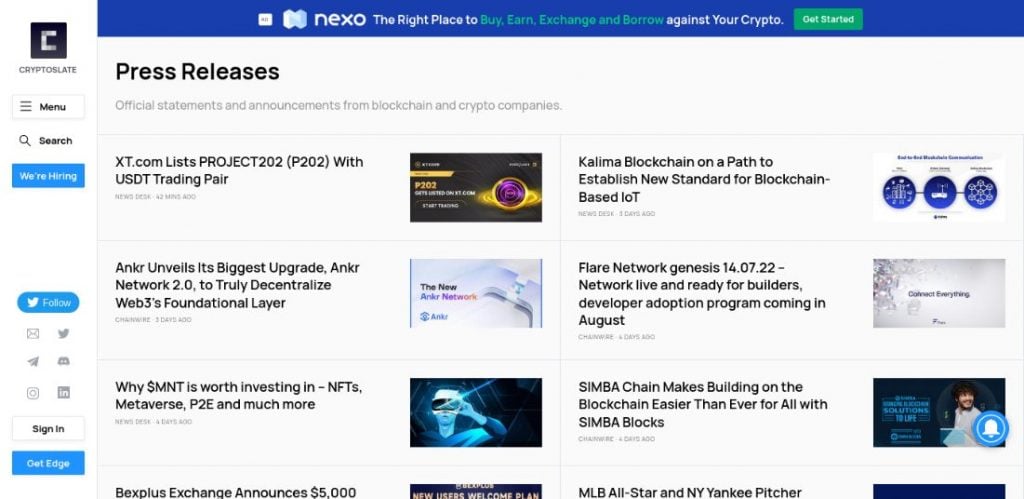This is a digital image from my website, NextO—your ultimate destination to buy, earn, exchange, and borrow against your crypto assets. Prominently featured is a "Get Started" button inviting users to engage with the platform. Below this, a series of press releases are showcased, offering initial statements and announcements from various blockchain and crypto companies.

The highlighted news includes XT.com's listing of Project 202 with a USDT trading pair. Another significant update is ANKR's most substantial upgrade, unveiling ANKR Network 2.0 aimed at truly decentralizing Web3's foundational layer. Furthermore, there is an emphasis on YMNT as a valuable investment opportunity in NFTs, the Metaverse, Play-to-Earn (P2E), and more. Additionally, BIX Plus exchange announces an enticing offer of 5,000 units. The latest titles do not stop there; Kalima blockchain is presented as being on a promising path to establish a new standard for blockchain-based Internet of Things (IOT) solutions.